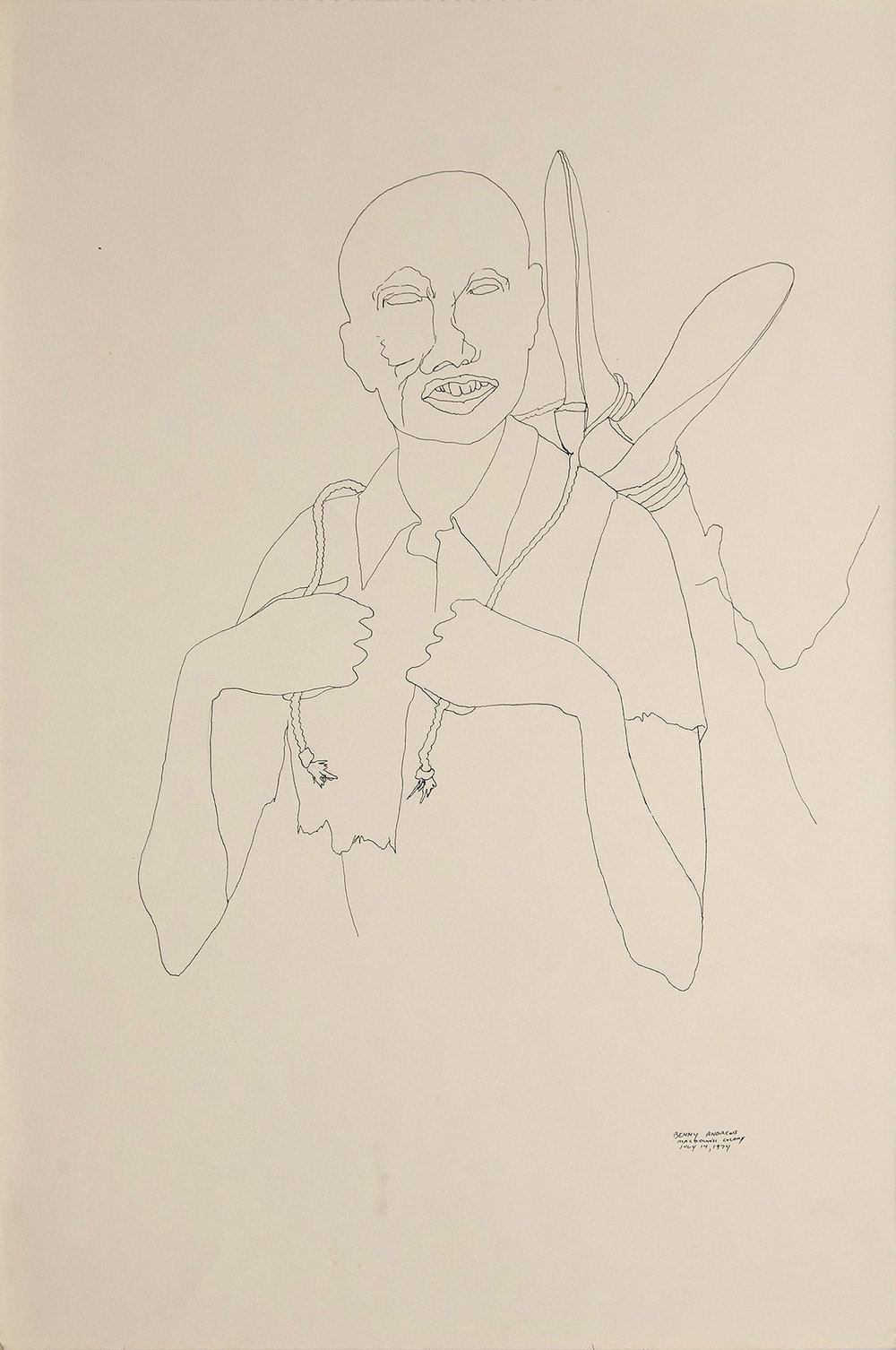This sketch, rendered on a light beige, canvasy paper, features a bald man with a solemn expression and no pupils in his eyes. He has a crooked nose, large crooked teeth, and a visible scar on his cheek. The man is wearing a button-up shirt with cut-off sleeves and is gripping a rope over his shoulders, bent at the elbows. This rope is tied to a pair of bound feet, which appear propped over his shoulders, suggesting he is dragging someone, likely a woman. The feet are in long dress shoes, and the legs extend out of view, blending into the background. The drawing is very simple and lacks detail, being a basic line sketch. In the bottom right corner of the sketch, there is an indistinct signature, possibly reading "Benny Anderson" with an unreadable date.